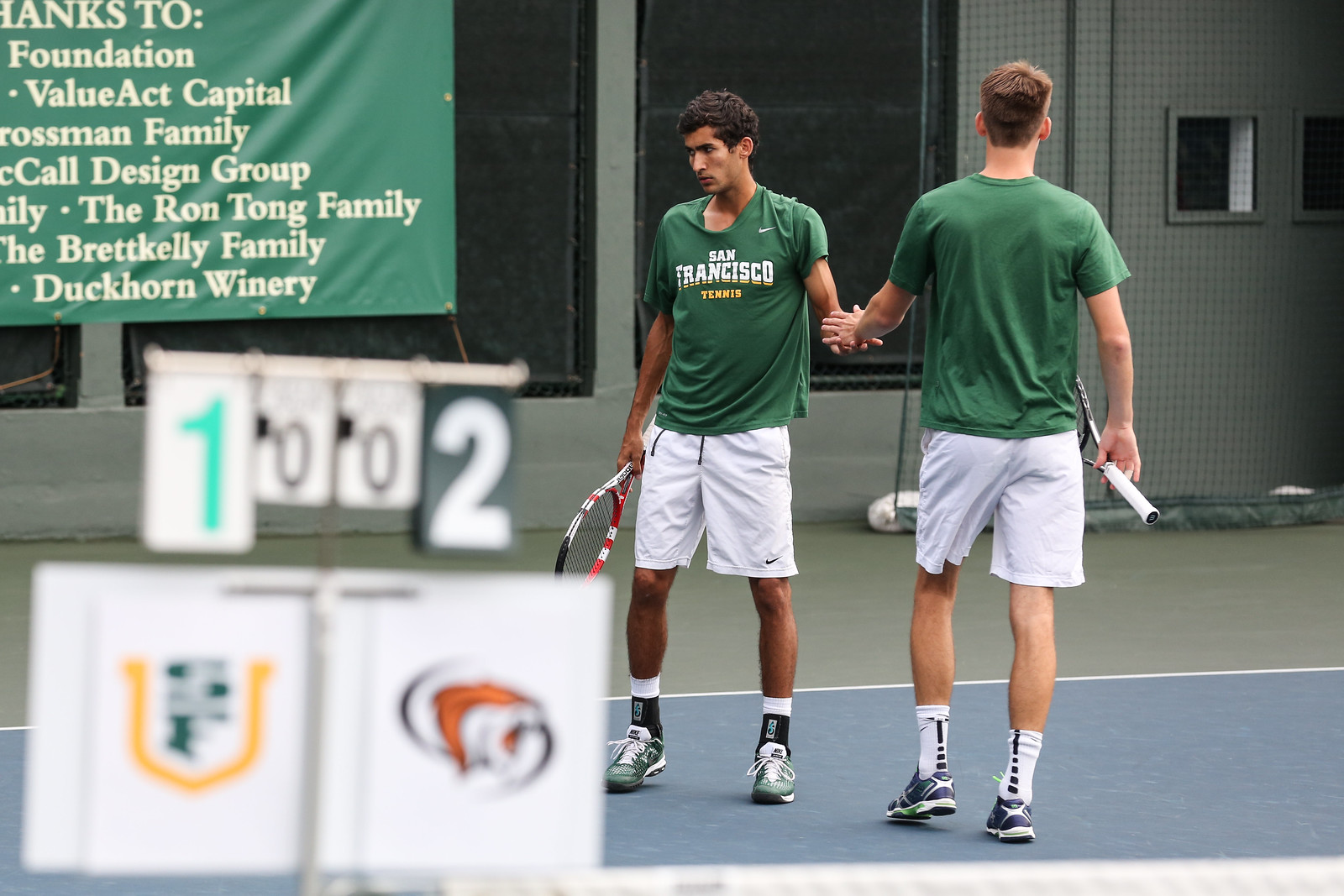The image captures a doubles tennis match, with two players standing side by side on a tennis court, both holding tennis rackets. They are clad in matching green t-shirts and white shorts; the t-shirts bear the text "San Francisco Tennis." The player on the left, facing the direction of the camera, appears to be engaged with his teammate in what seems like a high five, his expression intense and focused. Behind them, the backdrop features several sponsorship banners partially captured in the frame. These banners mention sponsors such as "The Ron Tong Family," "The Brett Kelly Family," "Duckhorn Winery," and "Value Act Capital," among others. In the blurred foreground, there's a scoreboard displaying the numbers "1002," but its significance remains unclear. Additionally, a few logos can be seen in the lower left-hand corner, though they are out of focus.